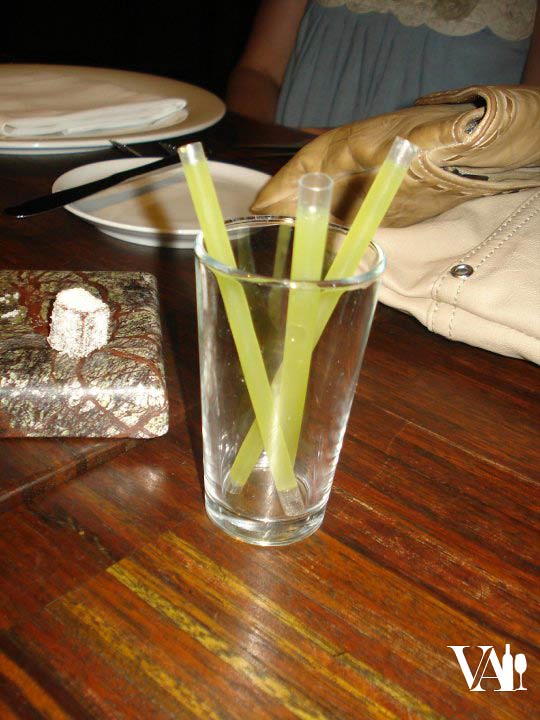The image showcases a detailed scene at a restaurant. Central to the image is a clear plastic glass containing three straws filled with a yellowish substance, likely resembling lemon juice or another citrus drink. This glass sits on a brown wooden table with a glossy finish. To the left of the glass is a plate featuring a white-frosted cube, possibly a dessert item. Surrounding the glass, a white plate is visible with a silver knife resting on it, accompanied by additional plates, utensils, and a napkin in the background. Behind the glass, several purses can be seen, including a white and light brown leather purse. In the bottom right corner of the image, a logo with the letters "VA" is displayed, along with symbols of a wine bottle and glass. Additionally, in the background, a person wearing a blue shirt and visible arm suggests the presence of restaurant patrons.